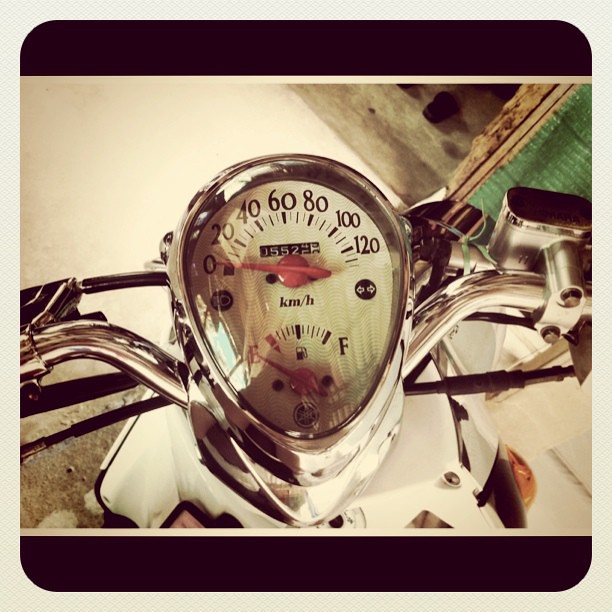This sepia-toned image captures a vintage speedometer and fuel gauge of an old motorcycle or scooter, encased under an oval-shaped, slightly bulbous glass dome. The speedometer, calibrated in kilometers per hour, has markings that reach up to 120 km/h. The accompanying fuel gauge displays an empty reading. Only the gauges, a segment of the chrome handlebars, and a portion of the vehicle’s white bodywork are visible in the photograph. Notably, a green thread is tied around the handlebar, adding a unique detail to the image. The speedometer features a classic, retro font, and the odometer shows a mileage of approximately 150,000, 155,000, and 250,000 kilometers. Two horizontal black lines are present at the top and bottom of the image, framing the scene. Despite its vintage appearance, the sepia filter suggests that this may not be an actual old photograph but a modern image edited to evoke a nostalgic feel.